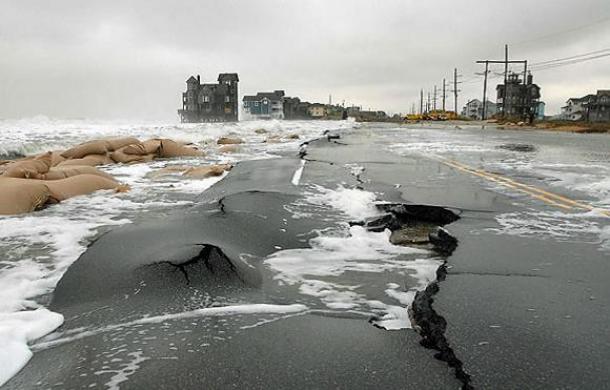The image captures a storm-battered road that has suffered severe water damage, rendering it undriveable. Ocean waters have breached sandbag barriers, causing extensive flooding and leading to the asphalt on the road to crack and buckle dramatically, as if struck by an earthquake. The road, which features a prominent yellow centerline, is slick with moisture from the wave action rather than recent rain. To the left side, large sandbags lie futile against the encroaching sea.

In the background, sizable beachfront homes sit surrounded by water, extending hundreds of feet past the properties, indicating a significant flooding event. The left side appears completely affected, with those houses evacuated due to the rising waters. The horizon shows a series of power line posts receding into the distance, reinforcing the desolation and the impact of the storm. The sky is overcast, adding to the dreary atmosphere. The scene is a stark display of nature's force, leaving a once-clear roadway in a chaotic, unpassable state.